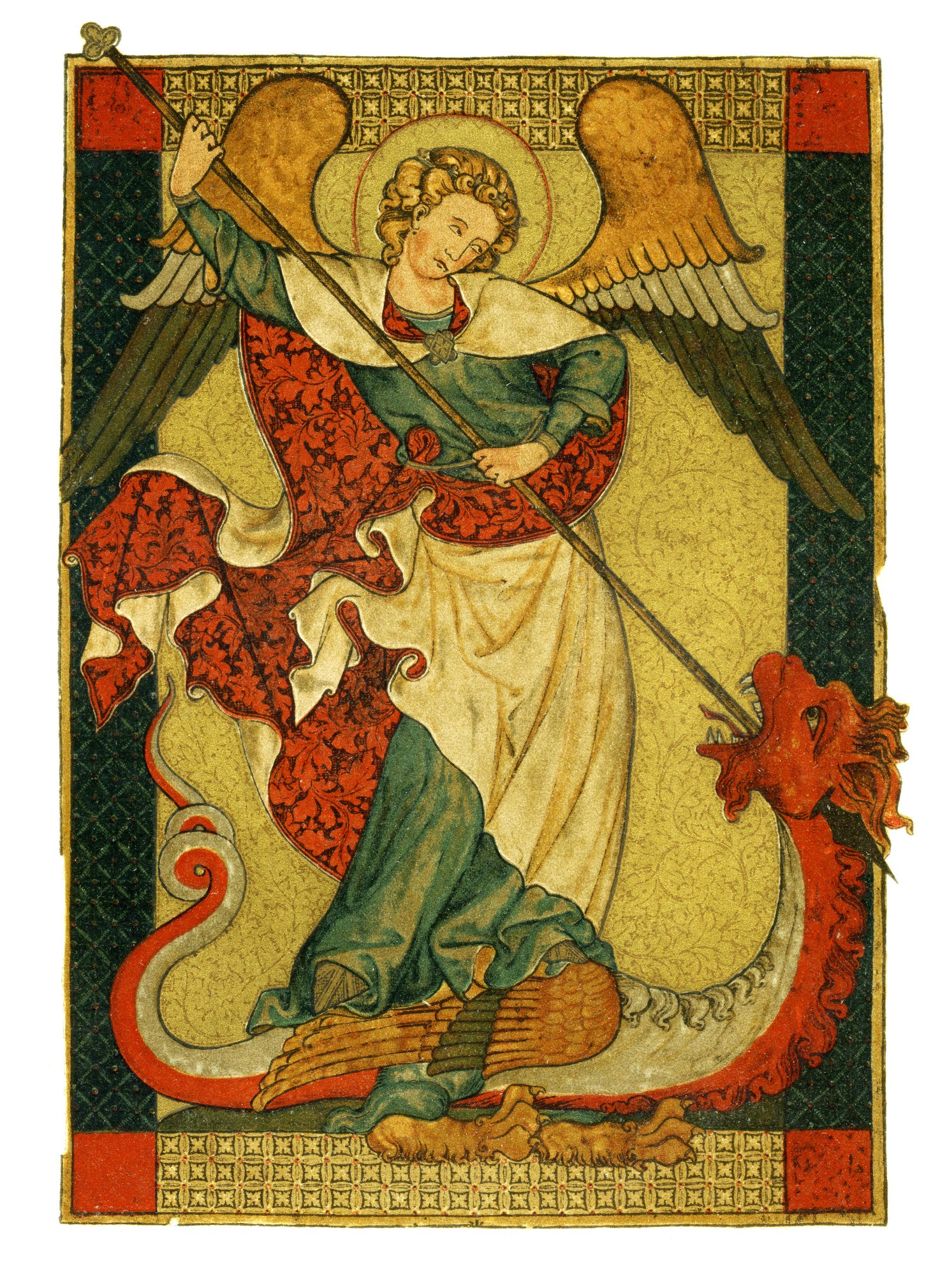This illustration, likely from the medieval or Renaissance period, depicts a dramatic and vivid religious scene. At the center stands an angel, possibly Saint Michael the Archangel, adorned in a white robe with green and red elements, and distinguished by a radiant halo surrounding their head. The angel's yellowish blonde, medium-length curly hair flows around their face, and their large, stately wings extend prominently from their back. The angel exudes a calm but determined presence as they wield a spear, driving it forcefully into the open mouth of a red dragon-like demon. The demon, with a serpent-like appearance, snake-like tongue, and a coiled tail, lays defeated on its back with its head raised in a final struggle. The artwork is devoid of other figures, animals, buildings, or modern elements, focusing solely on the intense confrontation between the celestial and infernal beings. The detailed depiction of the angel’s stance over the dragon emphasizes the triumph of good over evil in this visually compelling scene.